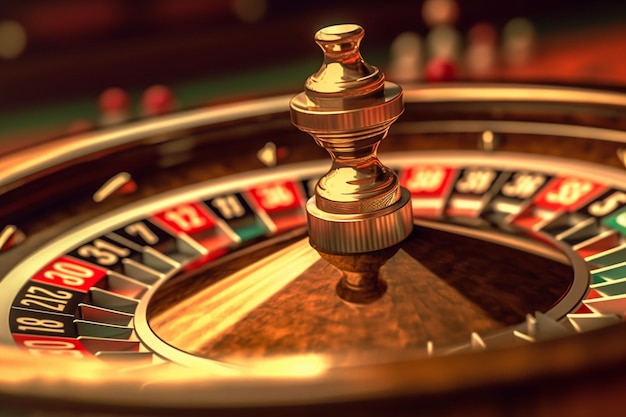This detailed, close-up image depicts a roulette table, as typically found in a casino. The focal point is a spinning roulette wheel featuring numbered slots in red, black, and green. The wheel's center boasts an ornamental gold spindle with a design reminiscent of a dumbbell, adorned with vertical lines for added texture. Around the outer edge of the wheel are numbered pockets where a white ball would land, with some numbers appearing unusual, such as an upside-down 2, suggesting the image may be AI-generated. In the background, there are blurry poker chips and other tables, reinforcing the casino setting. The overall scene has an exceptionally smooth appearance, contributing to the impression of being artificially created.